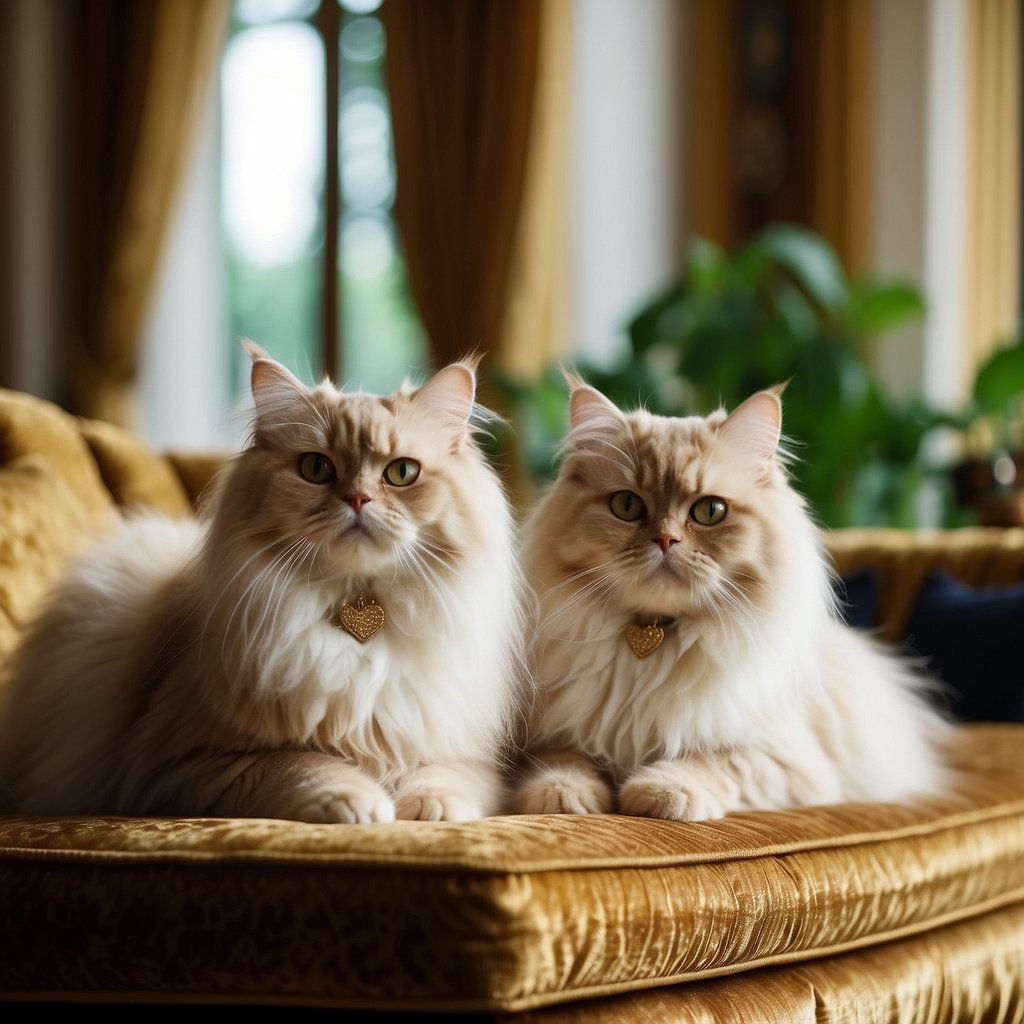This striking photo captures two nearly identical, long-haired cats with soft, fluffy, creamy goldish-beige fur. Their tufted ears and groomed manes add to their majestic appearance. Both cats are adorned with golden heart lockets on their collars and have enchanting greenish eyes that stare directly into the camera, giving the impression of a perfectly synchronized, almost AI-generated image. They are perched gracefully on their front paws atop a luxurious, gold crushed velvet upholstered sofa. The cozy setting features dark navy blue pillows, potted plants, and a window with thick, ornate golden curtains in the background. The room exudes a sense of elegance and sophistication, complementing the cats' equally regal demeanor.